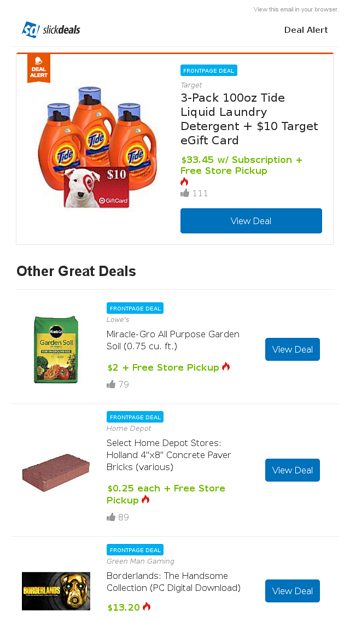**Slick Deals Email Notification**

**Top Deal:**
- **Deal Alert:** Three-pack of 100-ounce Tide Liquid Laundry Detergent + $10 Target Gift Card for $33.45 with subscription and free store pickup. 
- **Popularity:** 111 thumbs-up
- **CTA:** [View Deal] (Button in blue with white font)

**Other Great Deals:**
1. **Miracle-Gro All-Purpose Garden Soil (0.75 cu. ft.):**
   - **Price:** $2.00
   - **Availability:** Free store pickup
   - **Popularity:** 79 thumbs-up
   - **CTA:** [View Deal] (Button in blue with white font)

2. **Select Home Depot Stores - Holland Concrete Paver Bricks (4×4×8, various colors):**
   - **Price:** $0.25 each
   - **Availability:** Free store pickup
   - **Popularity:** 89 thumbs-up
   - **CTA:** [View Deal] (Button in blue with white font)

3. **Borderlands: The Handsome Collection (PC Digital Download):**
   - **Price:** $13.20
   - **CTA:** [View Deal] (Button in blue with white font)

**Header Details:**
- **Deal Alert:** Orange line with Deal Alert text on the left.
- **Browser Option:** "View this email in your browser" in light gray at the top.